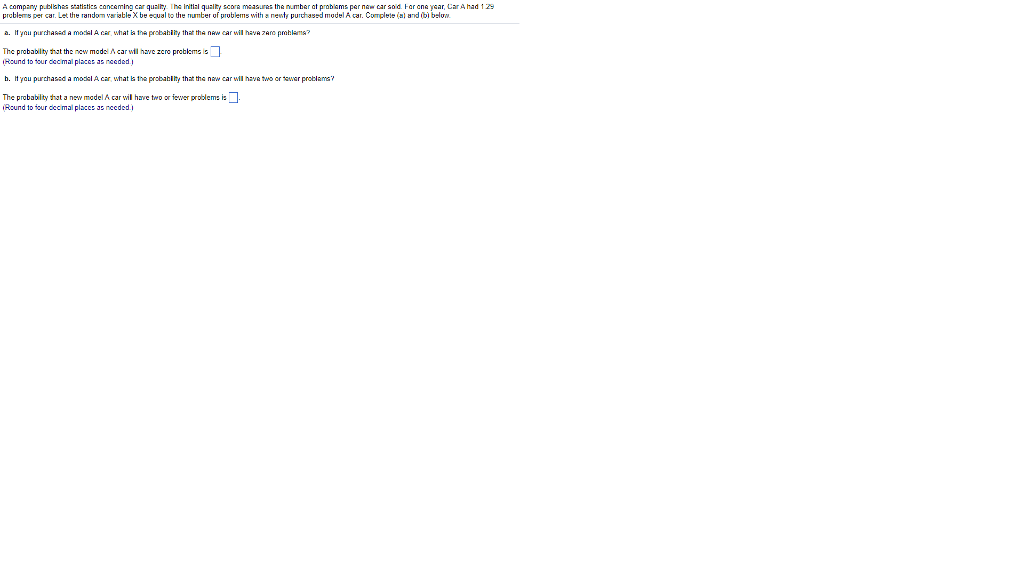This image is a screenshot of a typed question on a white background, with black text. It presents a question related to car quality statistics published by a company. The question revolves around the initial quality score, which measures the number of problems per new car sold. Specifically, the focus is on model A cars, which had an initial quality score of 29 problems per car in one year. 

The screenshot defines the random variable \(X\) as the number of problems with a newly purchased model A car and includes two parts to be completed: 
- Part A asks: "If you purchased a model A car, what is the probability that the new car will have zero problems?" Below this question, there is a box to input the probability, followed by instructions in blue text that read: "(Round to four decimal places as needed.)"
- Part B asks: "If you purchased a model A car, what is the probability that the new car will have two or fewer problems?" Below this question, there is an answer box, with similar blue text instructions: "(Round to four decimal places as needed.)"